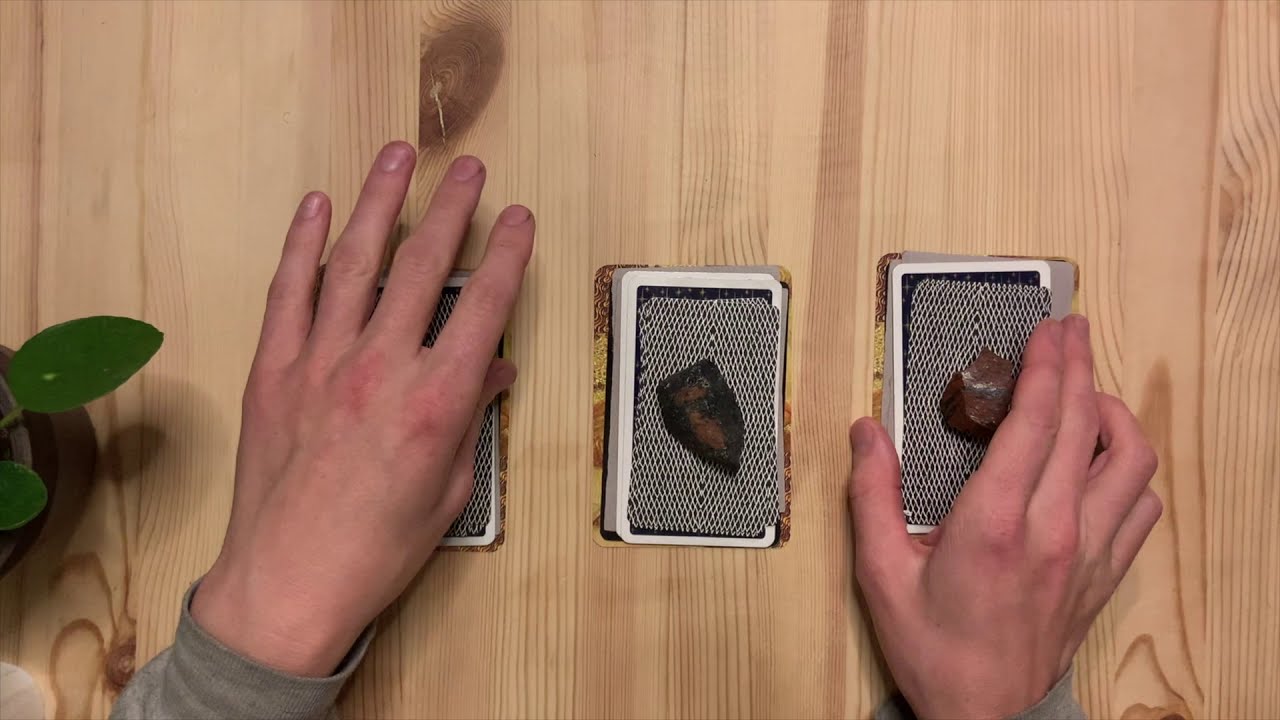In this overhead photograph, we see a light-colored wooden surface, likely a table, showcasing three distinct stacks of cards arranged horizontally across the image. The wood appears unfinished, presenting a natural grain pattern. There are two human hands visible; the left hand extends over and almost covers the first stack, while the right hand grasps the third stack. Each hand belongs to a person wearing a long-sleeved gray top, from which a gray wristband is discernible. 

Each stack of cards has a unique object on top of it. The left stack is nearly obscured by the left hand, leaving its contents ambiguous. The middle stack features a small black rock placed on the cards, while the right stack has another rock, also black, resting on top. The cards themselves possess a black and white design and are placed on top of slightly larger mats. 

In the upper left corner of the image, a potted plant with a few green leaves adds a touch of natural greenery to the scene, enhancing the earthy wood grain background which integrates well with the overall aesthetic.